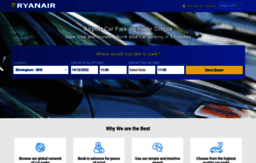The image appears to be a very small, possibly a screenshot of a low-resolution website, making the text blurry and difficult to read. In the upper left corner, the word "Ryanair" is displayed in white letters against a blue background. Next to it, on the left side, there is a small yellow icon, presumably a logo. In the background, faint images of cars suggest that the website might be related to either purchasing flights or renting cars, though this context is unclear due to the resolution. Below this area, there are various input fields, possibly intended for selecting states or cities, although the specific details are indistinguishable. The overall background is predominantly blue with the outlined silhouettes of cars embedded within the design.